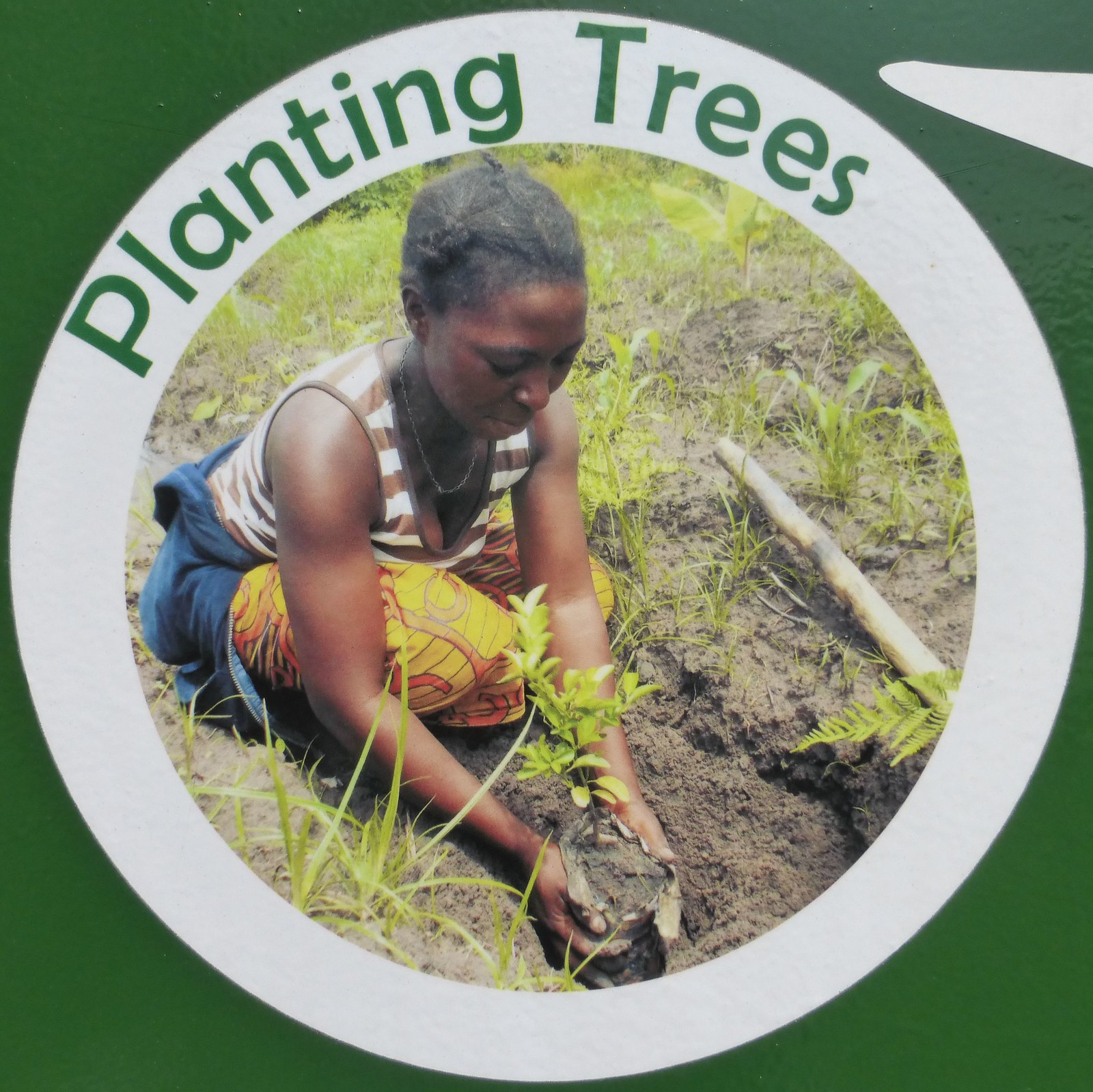The image portrays an advertisement poster with a green background framed by a green square. Inside the square is a large white circle, bordered by the green text "Planting Trees" at the top. Central to the image is a photograph of a woman squatting on a muddy, grassy ground as she plants a tree sapling into a small pit. The woman, adorned in orange and yellow pants, a sleeveless brown and white striped t-shirt, and a silver chain necklace, has a blue coat or shirt wrapped around her waist. In her hands, she holds a mound of dirt enveloping a twig-like sapling with multiple leaves. To the right of the woman, a wooden-handled shovel is partially visible, grounding the scene in the activity of tree planting.